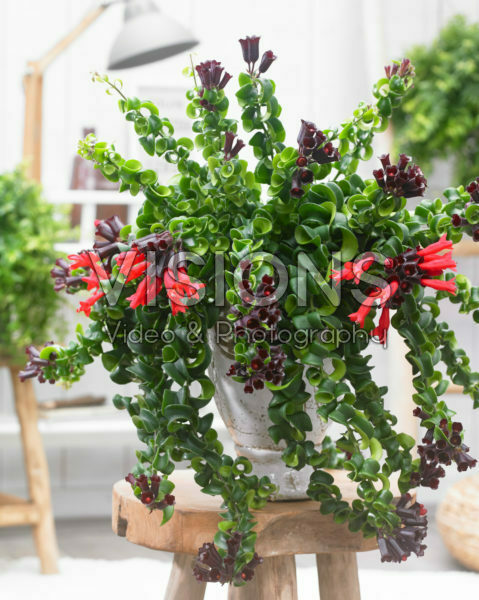The image captures a close-up shot of a green plant adorned with small purplish buds and reddish-pink flowers on the verge of blooming. The plant is housed in a white ceramic vase with subtle gold speckles and sits atop a light wooden stool with a thick, round top. The stool appears to have four legs though only their tops are visible. Superimposed across the greenery in an almost opaque white font is the text "Visions, Video and Photography." The background features a white wall with an overhead conical white lamp. To the right, a blurred hanging plant can be observed, while another green plant on a similar wooden bench is also visible. A window with an external structure provides a glimpse of the outdoors to the left. The setting includes additional wooden structures holding various plants, contributing to a natural and serene ambiance.